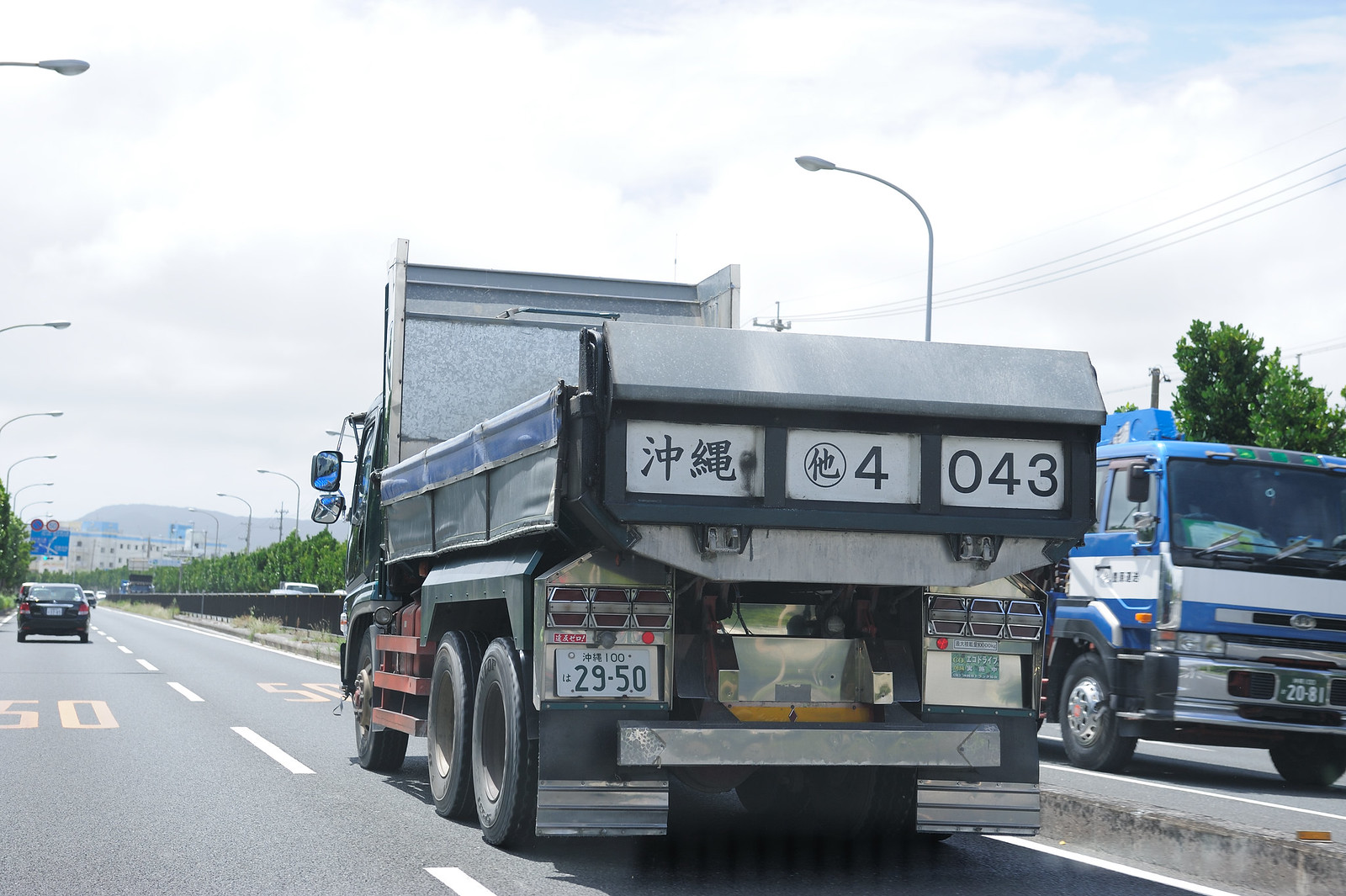In this photo, we see a busy four-lane highway under a predominantly cloudy sky with hints of blue in the upper right-hand corner. The highway features neatly marked white lines and concrete surfaces, with speed limit signs indicating 50, either in kilometers or miles per hour. Vehicles are driving on the left side of the road, suggesting a location in a foreign country. Green trees line the sides of the highway, and curved lampposts arch above the traffic. 

Prominently, we are positioned behind a large dump truck moving away from us, displaying Chinese characters and the numbers 4043-2950 on its rear door. The truck is a substantial ten-wheeler, easily identifiable by its silver bumper and black flaps edged with silver. A blue and white truck of similar size is seen heading towards the camera in the opposite lane, with a green license plate reading 2081. Additionally, there's a small car in the adjacent left lane ahead of the dump truck, contributing to the overall dynamic scene.